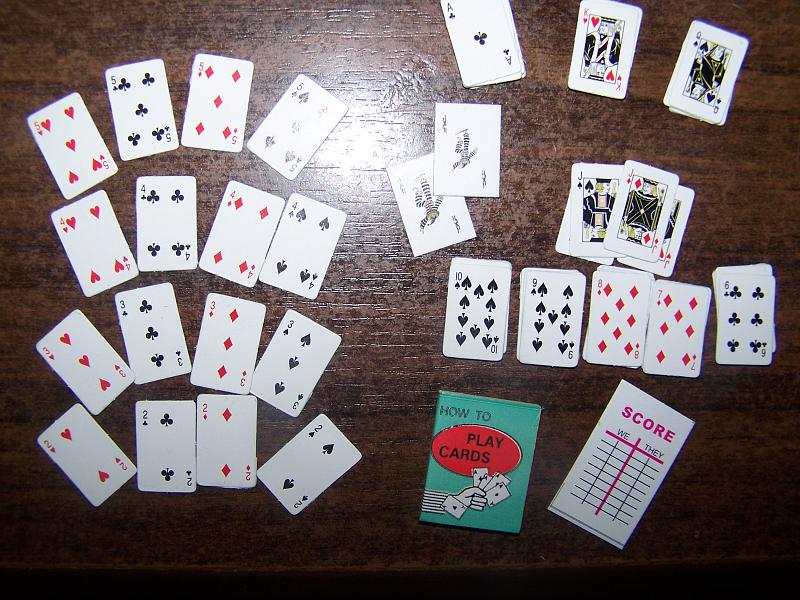An overhead color photograph showcases an assortment of playing cards meticulously arranged on a wooden surface, revealing the natural wood grain and a soft glare from a light source near the upper center. On the bottom right-hand corner, a rectangular, white scorecard, tilted slightly to the right, displays the word "Score" in red at the top, and below it, columns labeled "We" and "They." To the left of the scorecard, a small aqua green booklet titled "How to Play Cards" features a black-and-white cartoon illustration of a hand holding cards, with a red oval enclosing the words "Play Cards."

The deck of cards is neatly laid out on the table, organized by rank and slightly curved in rows. On the left side, there is a row of all the fives, followed by rows of fours, threes, and twos. In the top right corner, separate piles of aces, kings, and queens are neatly stacked. Below these, two overlapping jacks are placed, followed by a pile of jokers. Further below are individual stacks of tens, nines, eights, sevens, and sixes, completing the well-ordered array of playing cards.